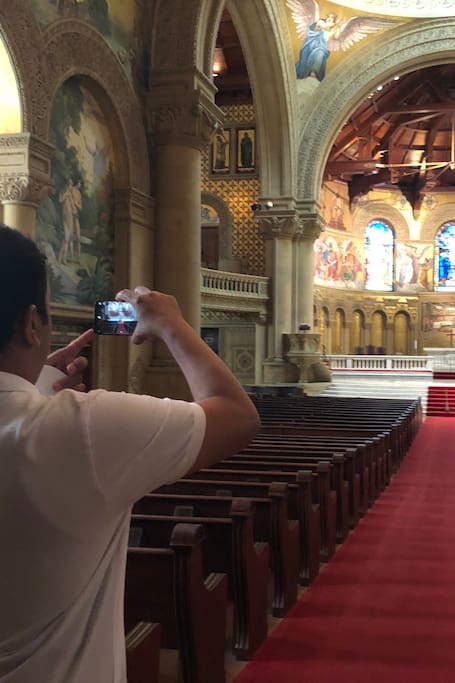The image showcases the ornate interior of a church captured from the left side. In the foreground, a man with short black hair, who appears to be either Caucasian or Hispanic, stands in the aisle wearing a short-sleeve white polo shirt. He is holding up his phone in his right hand, capturing a video or picture of the front of the church. To his left are rows of empty brown wooden pews. The aisle is adorned with a long red carpet leading down to the main altar area, where red steps ascend to the stage.

The background reveals a series of arches set against a lavish gold wall, adorned with religious decorations and intricate sculpting designs on the columns and outer walls. Larger arches above host ornate blue stained glass windows. The dome-shaped ceiling above is framed with visible wooden beams, contributing to the church's grandeur. Notably, behind the altar, there is a Renaissance-style painting featuring an angel with outstretched wings wearing a blue dress, among other detailed artwork that enriches the space.